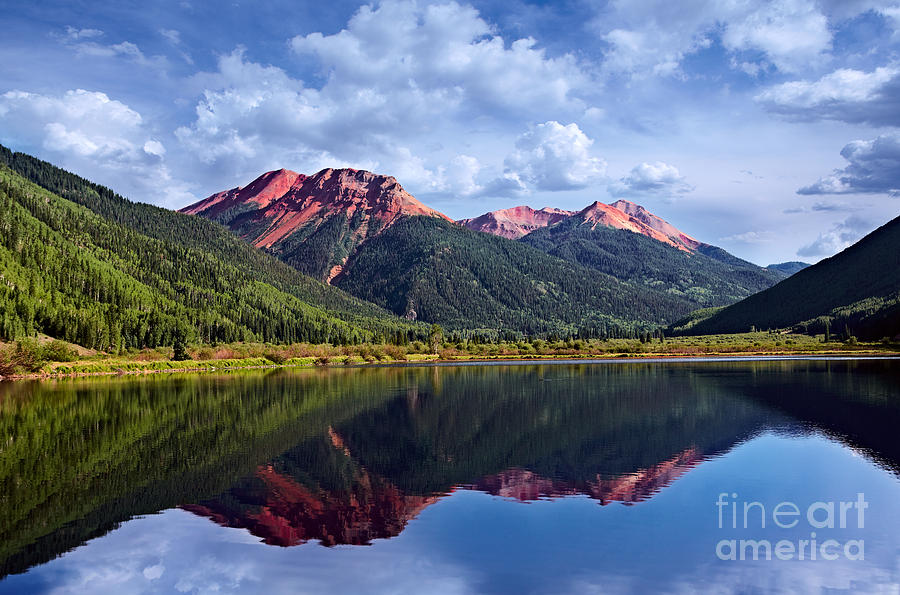This stunning professional fine art photograph, labeled "Fine Art America" in the bottom right-hand corner, captures a quintessential American landscape scene. The photograph features a picturesque mountain range with tall, tree-covered peaks and bare, rocky summits displaying red, brown, and pink hues. These majestic hills form a captivating backdrop to a serene, crystal-clear lake that perfectly mirrors the surrounding mountain scenery.
 
The sky above is a flawless blue, dotted with fluffy white clouds that add to the scene's tranquility and beauty. Sunlight bathes the mountain peaks and partially illuminates the lake, enhancing the visual appeal. The entire composition exudes a sense of pure, untouched wilderness, making it an ideal representation of America's natural splendor, a view you’d expect while envisioning or visiting the quintessential American landscape. The absence of human figures emphasizes the pristine beauty of this magnificent natural setting.